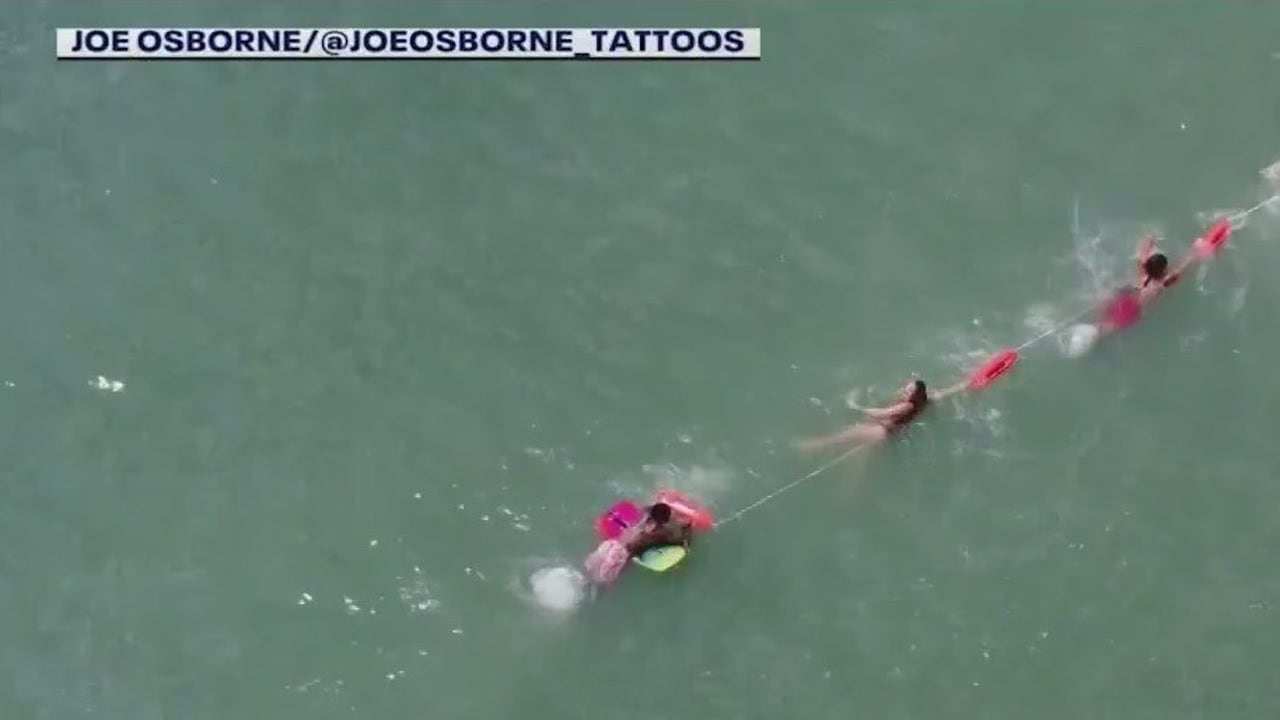This aerial drone photograph, presented in a wide horizontal landscape orientation, captures three individuals swimming in a calm, light greenish-blue ocean. Viewed from above, the image showcases a diagonal alignment of swimmers tethered by a white rope. Each swimmer holds onto a red-orange flotation device, suggesting a buoy line. 

The person at the bottom center of the image, with long dark hair and wearing swim attire, appears to be lying on a pink and green floatation device, periodically glancing back at the others. Midway along the rope, another swimmer is visible, and a third swimmer is closer to the upper right edge of the picture. The water surface has a dark grayish tinge with tiny ripples. 

In the upper left corner, a white rectangle contains the text “Joe Osborne / @Joe Osborne tattoos,” likely an advertisement for a tattoo company. The overall sense is one of organized, perhaps assisted, movement through serene waters, with photographic realism emphasizing the naturalistic details of the scene.